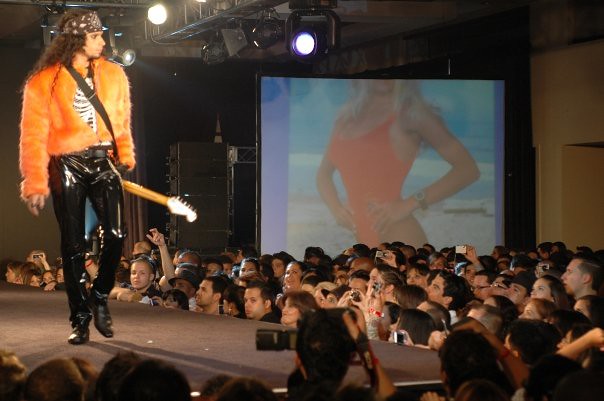The photograph captures a dynamic stage performance on a raised black stage, which extends from the bottom left to the bottom center of the image. A charismatic performing artist, possibly a rock star, stands on the left side of the stage adorned in a striking, big orange fuzzy coat over a shirt that appears to feature a skeletal rib cage design. His shiny, painted-on black leather pants and heeled boots complete his flamboyant look. He carries an electric guitar slung across his back, with only the neck visible as the rest is obscured. The artist, a white man with long dark curly hair and a black bandana incorporating a visor, gazes intently towards the right side of the image.

Surrounding the stage, a large crowd of predominantly middle-aged individuals directs their attention toward the performer, many holding up their phones to capture the moment. Adding to the visual spectacle, a projector screen on the left side of the background displays an image of a woman from the chin down, clad in a red bathing suit with blonde hair, standing confidently with her hands on her hips against a beach backdrop. The overall ambiance is highlighted by stage lights aimed at the performer, with dark curtains creating a dramatic setting typical of live musical performances.